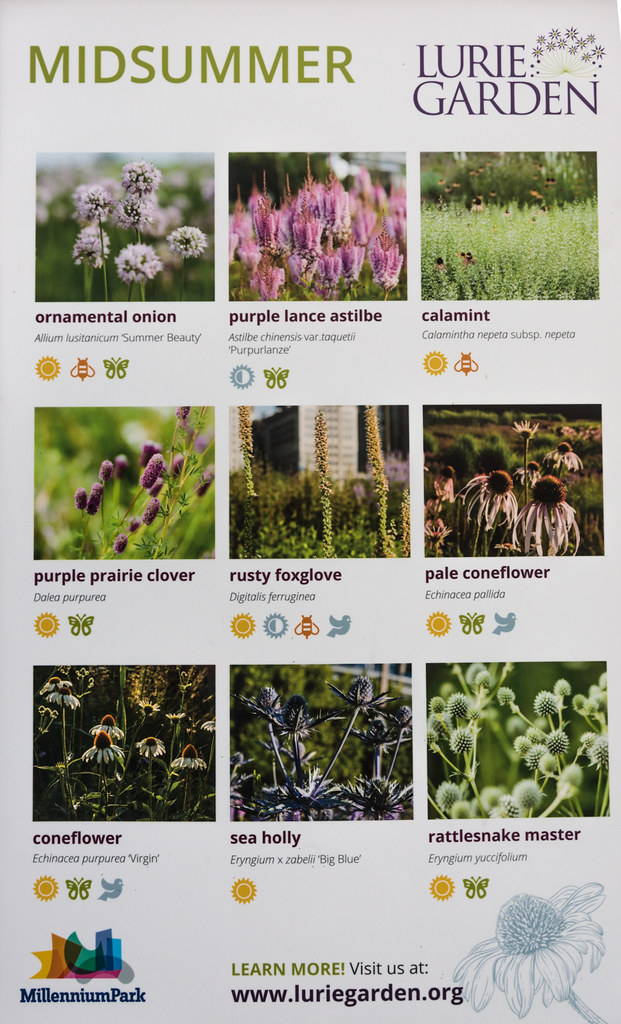This detailed poster, prominently displayed as part of Millennium Park's public offerings, showcases the diverse flora of the Lurie Garden. At the top, the poster features the title "Midsummer" in green letters, adjacent to "LURIE GARDEN" in bold, purple all-cap font. The layout consists of three rows, each containing three square photos of various plants, making a total of nine distinct images. These images are accompanied by detailed labels, though some text is too small to decipher fully.

The first row includes:
1. Ornamental Onion: Featuring fluffy, cloud-like white plants.
2. Purple Lance Astilbe: Displaying lavender-hued, slightly blurred flowers.
3. Calumet: Depicting white and green vertical branches.

The second row highlights:
1. Purple Prairie Clover: Small purple buds set against a green backdrop.
2. Rusty Foxglove: Tall, brownish, vertical plants.
3. Pale Coneflower: Wilted-looking purple flowers with a dark brown center.

The third row presents:
1. Coneflower: Similar to the Pale Coneflower, but with white petals and green surroundings.
2. Sea Holly: Unique dark blackish-blue petals.
3. Rattlesnake Master: Resembling cotton but with spikier textures.

At the bottom left corner, the poster features the Millennium Park logo. The color scheme for the entire poster includes vibrant shades of green, purple, blue, pink, and yellow. In the bottom right corner, there is a detailed drawing of a flower with a stamen. For more information, visitors are directed to "learn more, visit us at www.luriegarden.org", neatly positioned at the bottom of the poster. The overall design includes icons under each of the nine images, enhancing the educational aspect of this visually appealing and informative garden poster.